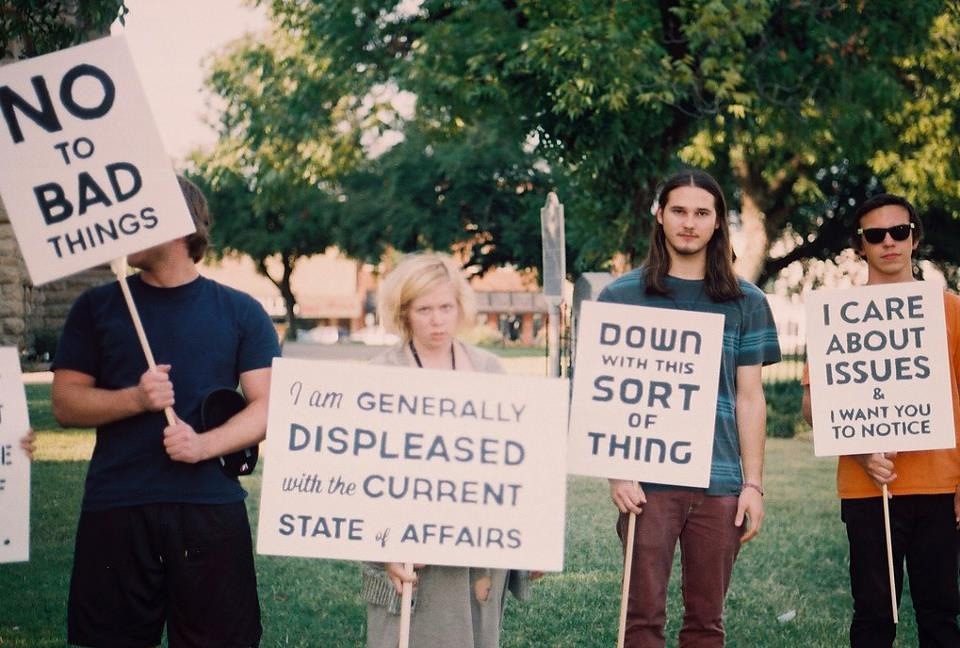In the image, we see a group of four young adults participating in a protest, standing in the center of a flat, grassy field. The scene appears to be set during the daytime in a downtown area, likely resembling the 1980s or 90s based on the image's coloration. The protesters, consisting of three men and one woman, are holding white picket signs with blue text, including messages such as "No to bad things," "Down with this sort of thing," "I care about issues," and "I want you to notice."

The individuals' attire is distinctly described: 

- **Man 1:** Wearing a blue shirt and looking away from the camera.
- **Woman:** In the center, with short blonde hair, a gray overshirt, and a dress, looking directly at the camera with a stern expression.
- **Man 2:** Next to the woman, with long black hair, a blue shirt with stripes, and red pants.
- **Man 3:** On the far right, wearing an orange shirt, black pants, and sunglasses.

Behind the group, there are trees with abundant leaves and several buildings, enhancing the depiction of a protest taking place in an outdoor, urban park setting. The colors in the image are vivid and varied, including black, white, dark blue, orange, green, tan, and brown.